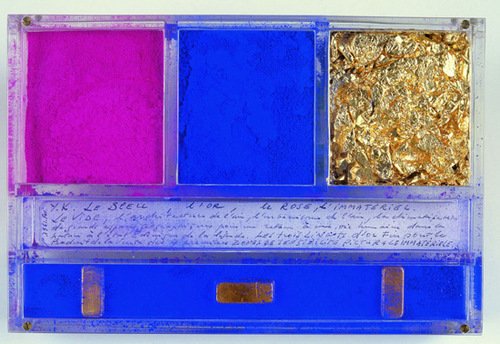The image depicts a horizontally aligned rectangular palette set against a subtle gray background, which almost creates a border around the colorful content. At the top of the palette, there are three square compartments filled with different materials: the left one contains purple (possibly paint or clay), the middle one is filled with blue, and the right one has irregularly shaped chunks resembling gold-colored foil. Below these squares, there is a thin rectangular section featuring a white piece of paper with blue, calligraphy-like writing in a language other than English. This appears to add a decorative or informative element to the palette. Further down, a wider rectangular section of the palette appears with a predominantly blue hue and contains three metallic pieces—two vertically aligned and one horizontally aligned—covered partially in blue and gold colors. The entire palette is encased in what seems to be a clear Lucite material, secured with four screws at the corners, giving it a display-quality finish.